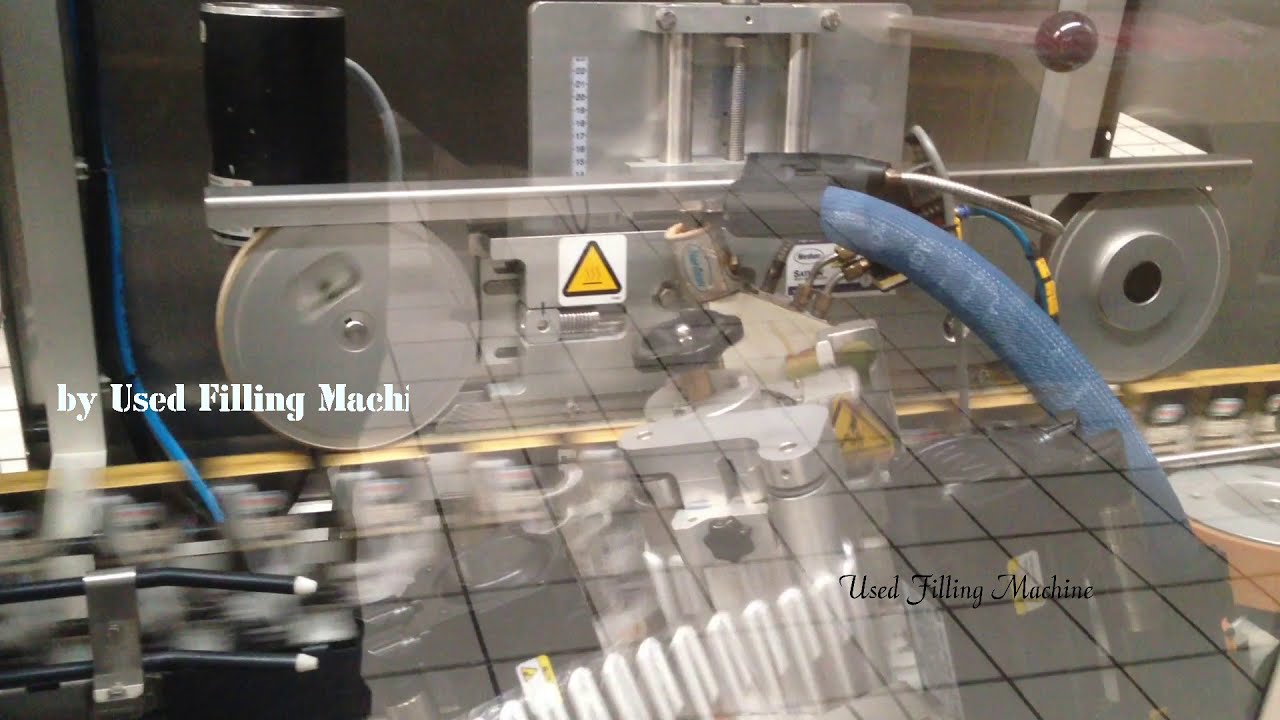This is a horizontally oriented, color photograph depicting advanced laboratory machinery predominantly composed of chrome and silver materials. The central machine features two prominent round components on the left and right sides, connected by a blue hose extending downward. On the left side of the image, partially obscured text in white reads, "By Used Filling Machine," although only "B-Y, Used Fillin Mach" is clearly visible. The photograph also shows part of a red stone tile floor peeking out on the right side. Additionally, a second set of text in black at the bottom right of the image repeats, "Used Filling Machine."

A notable feature of the image is an overlay effect, creating a photo collage that blends a transparent view of another piece of equipment into the scene. This secondary piece appears silver with a black dial, white swab-like vertical sticks, and a turnable valve. The collage adds a slight blur to the middle and lower parts of the image, contributing to an overall sense of depth and layering. The background colors are predominantly silver and black, enhancing the industrial ambiance of the photograph, which embodies a style of modern industrial commercial photography.